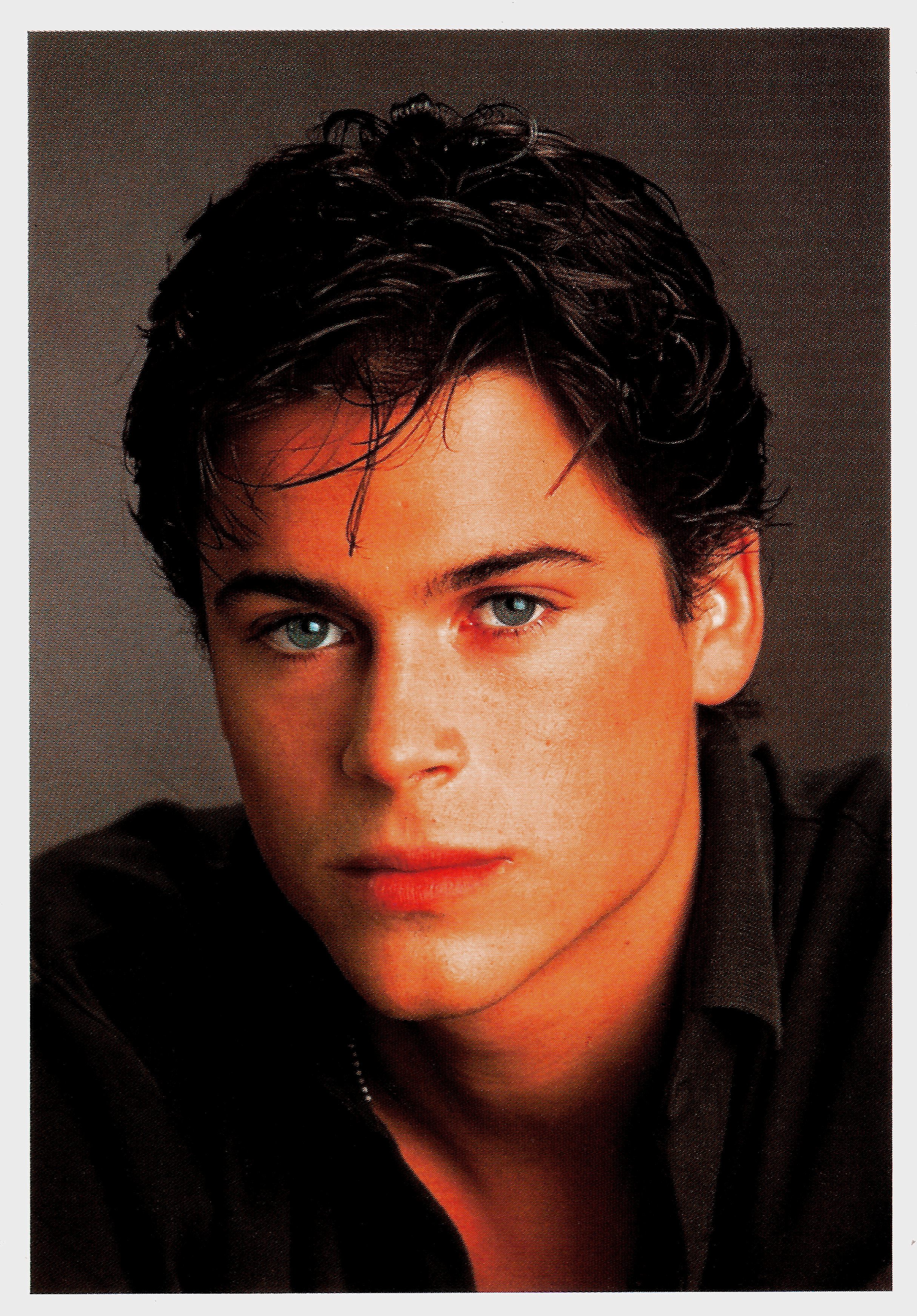This professionally taken headshot photograph features a young man, likely in his early 20s, positioned against a light gray solid wall. The image is framed by an even lighter gray border. The background appears slightly grainy, introducing a subtle texture. The man is wearing a black button-up shirt with multiple top buttons undone, though there was some mention of brown in descriptions which may be due to color perception variances. He has dark, intentionally messy hair and striking blue-green eyes. His well-groomed, dark eyebrows are notable, and he is staring directly into the camera with a stern, serious expression without a smile. There is a hint of a necklace visible at the corner of his neck. Some have speculated he resembles actors like Rob Lowe or Emilio Estevez, suggesting a familiarity with his appearance.